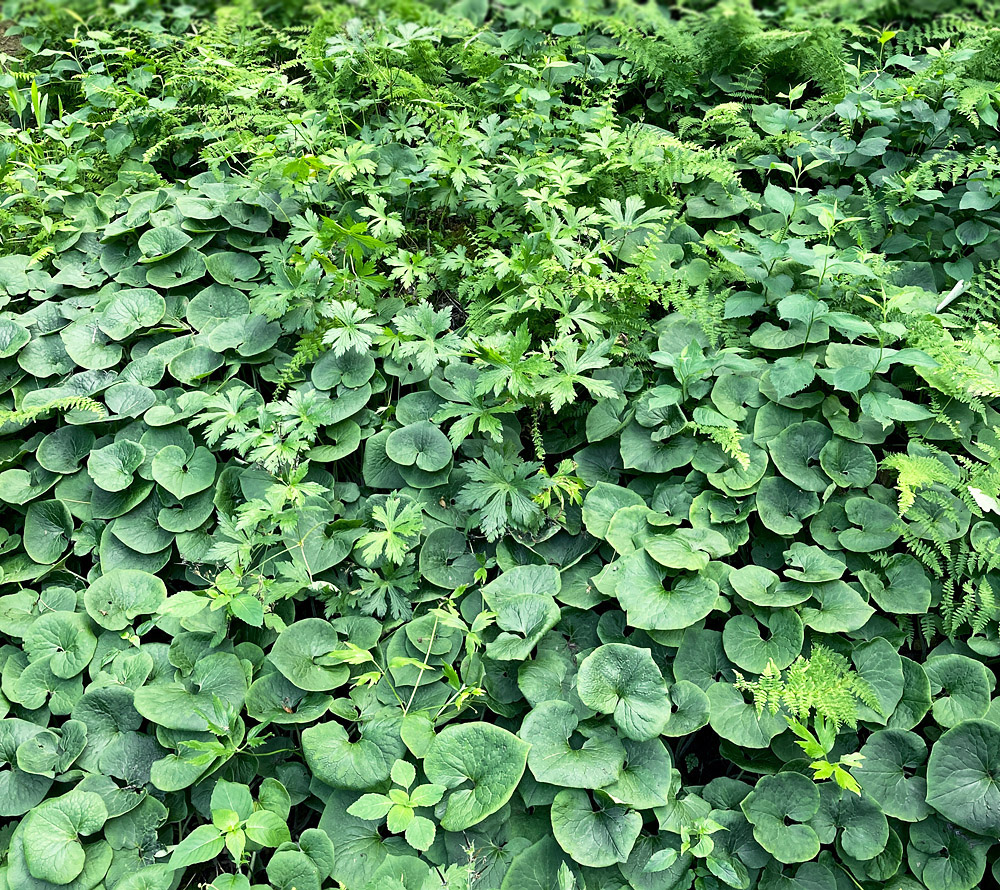The image captures a lush, dense field dominated by various types of greenery. Among the most prominent are vibrant green clovers with smooth, heart-shaped leaves, some with a light powdery topping. Interspersed with the clovers are ferns, characterized by their intricate, feather-like leaves, which appear in the bottom right and top sections of the image. Centrally located are plants with distinct five-prong shaped leaves adding to the variety. The field is a tapestry of different shades of green, ranging from deep, dark greens to lighter, brighter hues reflecting the sunlight. All the leaves appear smooth in texture, glistening under the light. The plants are so densely packed that the ground is entirely obscured, creating a seamless carpet of foliage that extends into the distance.